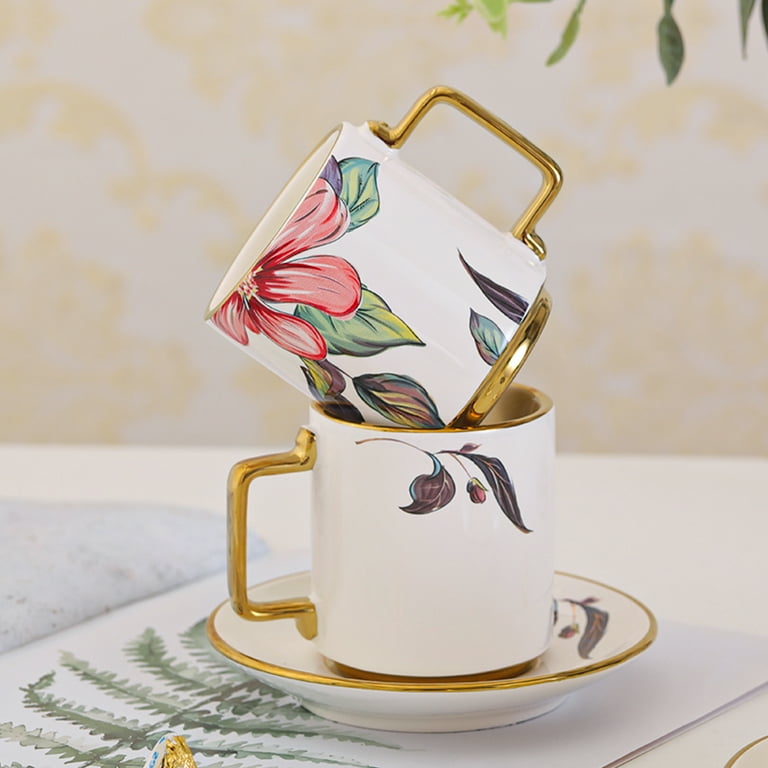This detailed photograph showcases two intricately decorated coffee cups placed on a table. The primary coffee cup rests elegantly on a matching saucer, both predominantly white adorned with plant motifs and bordered in gold. The cup on the saucer features two leaves and a delicate flower, and it is noted for its gold handle. 

Intriguingly, the second coffee cup is positioned at an angle, partially inserted into the first cup. This cup stands out with its more elaborate design, showcasing a red flower, green leaves, and additional decorative elements. It, too, is embellished with a gold handle, adding a touch of elegance.

The saucer, supporting the bottom cup, is set on what appears to be a placemat or tablecloth adorned with watercolor drawings of green leaves, lying on a table. The backdrop features a predominantly white wall with beige overtones, complemented by a hanging plant with a few leaves cascading from the upper right-hand corner, enhancing the serene setting.